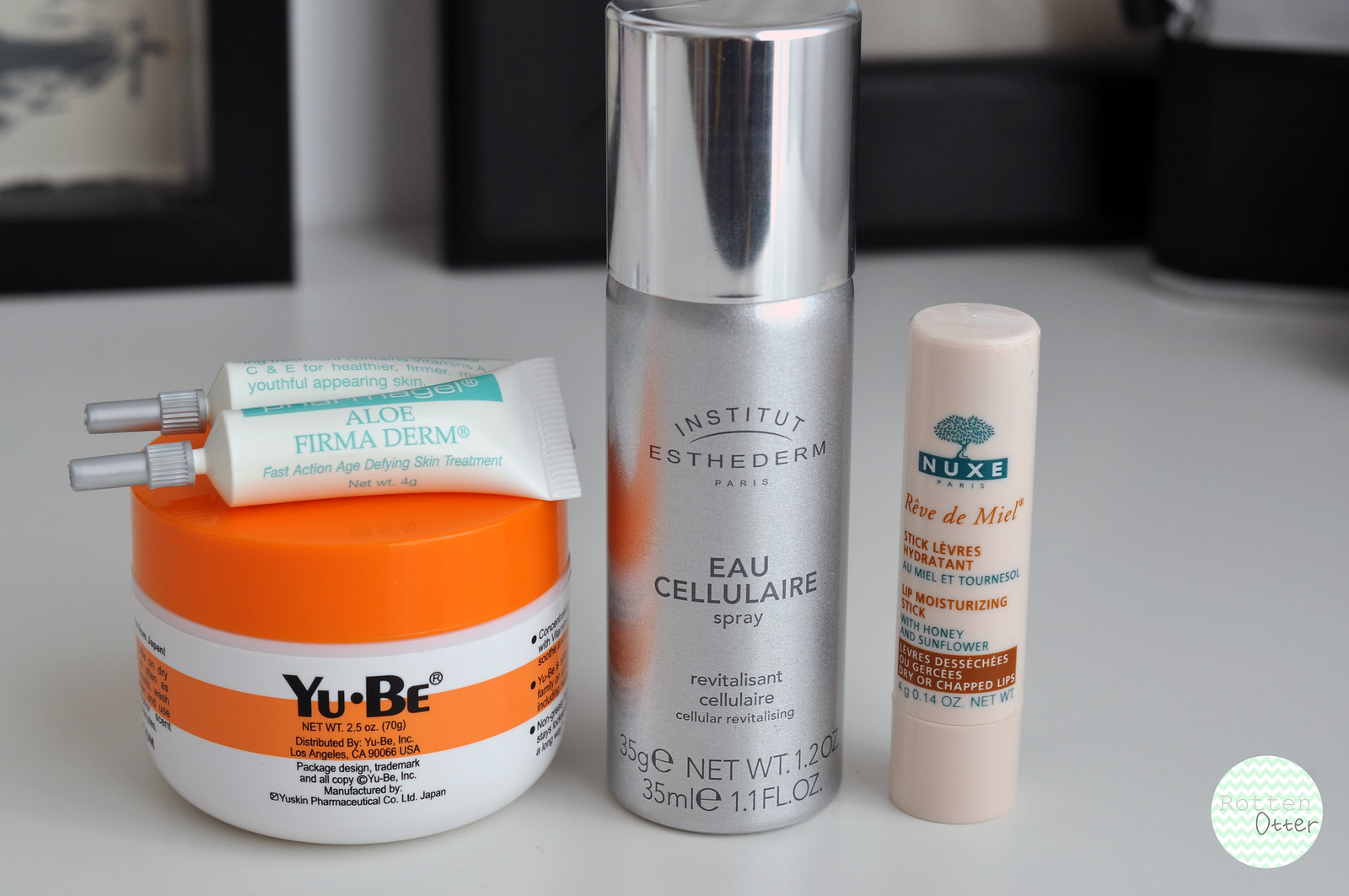This close-up photograph, likely taken with a high-resolution camera, captures an elegant display of five beauty products arranged on a pristine white cabinet. The products are centrally positioned in sharp focus, while the blurred background reveals indistinct picture frames, adding depth to the composition. In the bottom right corner, text reading "Rotten Otter" suggests the affiliation with a website or blog spotlighting these items.

The showcased products include: a cream from Yu-Be, identifiable by its distinctive white container with an orange lid; Aloe Firma Derm, a tube placed atop the orange lid of the Yu-Be cream; an Eau Cellulaire hydrating spray, prominently centered; and Rêve de Miel, a soothing chapstick by Nuxe, positioned on the right. Each product's packaging detail and brand are clearly visible, making this an informative and aesthetically pleasing depiction of skincare essentials.